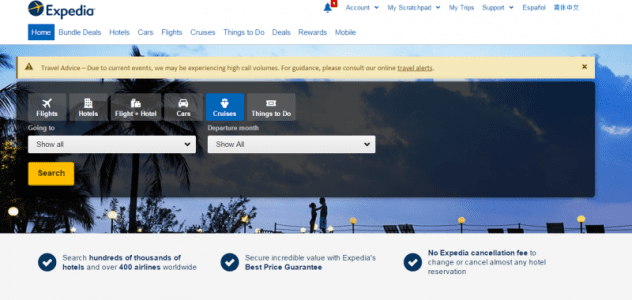This image showcases the Expedia homepage. Dominating the upper-left corner is the iconic Expedia logo, rendered in navy blue. Adjacent to the logo, a blue circle houses a yellow airplane icon. To the right, a blue notification bell is prominently displayed. The top navigation bar includes tabs for "Account," "Scratchpad," "My Trips," "Support," "Español," and several Japanese characters or symbols.

Directly beneath the Expedia logo lies another navigation strip featuring links to "Home," "Bundle Deals," "Hotels," "Cars," "Flights," "Cruises," "Things to Do," "Deals," "Rewards," and "Mobile."

Below these links, the page transitions into a serene blue sky background. A pop-up window appears, featuring icons for different booking categories: "Flights," "Hotels," "Flight + Hotel," "Cars," "Cruises," and "Things to Do." Within the pop-up, there are also two drop-down menus for "Destination" and "Departure Month," followed by a prominent yellow search button.

At the bottom of the image, three checkmark icons hint at the benefits and assurances provided by the service.